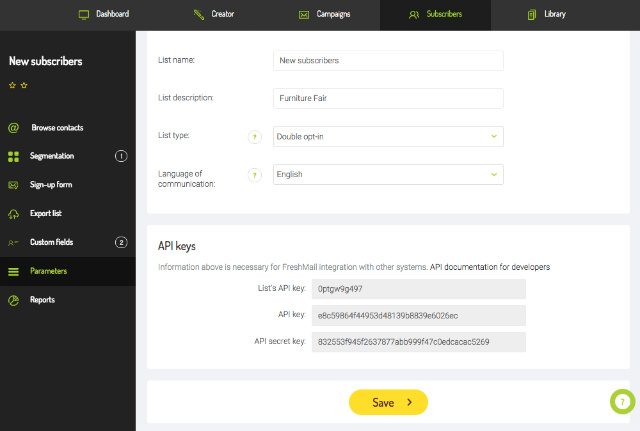The dashboard interface is divided into several key sections highlighted at the top, including "Creator," "Campaign," "Subscribers," and "Library." Beneath the main navigation, additional options are presented: "New Subscribers," "Browse Contacts," "Segmentation," "Sign Out Form," "Export," "List," "Custom Fields," "Parameters," and "Reports."

The interface includes fields such as "List Name," "New Subscribers," and "List Description" with an example entry labeled "Furniture Pair." Additional list-specific settings include "List Type," which is set to "Double Opt-in," alongside options for "Language and Communication." 

Furthermore, the dashboard provides API integration capabilities with the text indicating, "Information above is necessary for fresh file integration with other systems." The section labeled "API Documentation for Developers" offers various API keys required for system integration. Examples of these keys include:
- API Key: 0PTGW9G497
- API Key: EAT5986F449
- API Key: 538D48139BAA39E6026CC
- API Segment Key: 832553F945F263
- API Segment Key: 7877EBB999F47C0EDCACAC5269

Reiterated at the top is the list of sections: "Creator," "Campaign," "Subscribers," "Library," and "Library Pair."